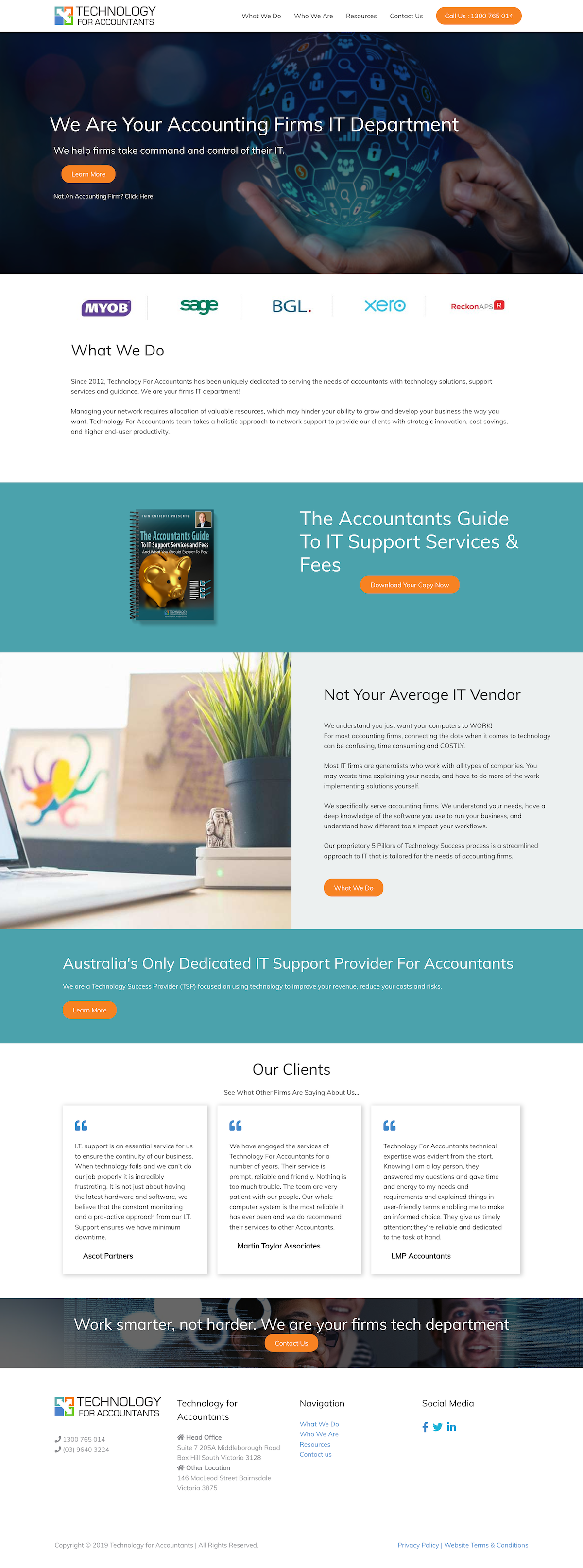Certainly! Here is a cleaned up and detailed version of the caption:

---

The image showcases a technology application designed specifically for accountants. At the top left, an icon featuring four colored squares (green, blue, and orange) with three arrows signifies its technology focus. The interface includes multiple tabs labeled "What We Do," "Who We Are," "Resources," "Contacts," and a contact number, "1-300-765-014." Below these tabs is a striking background image of a hand holding a globe, adorned with various IT-related icons such as settings, logs, and Wi-Fi signals. The globe itself has a captivating blue and purple hue.

Prominently displayed in front of the globe is the text: "We are your accounting firm IT department. We help firms take command and control of their IT," followed by a vibrant orange "Learn More" button. Just beneath this, an advisory states, "Not an accounting firm. Click here."

The subsequent section has a white background featuring logos of sponsors such as MYOB (purple), Search (green), BGL (blue), Xero (blue), and Reckon Apps (red and gray). Further down, the text reads: "What We Do: Since 2012, [Company Name] has been uniquely dedicated to serving the needs of accountants with technology solutions, support services, and guardianship." 

Details continue to describe their services: "We are your firm's IT department. Managing your network requires the allocation of valuable resources, potentially hindering your business's growth. [Company Name] takes a holistic approach to network support, providing clients with strategic innovation, cost savings, and heightened end-user productivity."

The final section on a blue background introduces a resource: "The Accountant's Guide to IT Support, Service, and Fees," featuring an image of a book available for download. It reads, "Download your copy now," in bold orange. Concluding the presentation, it states: "Australia's only dedicated IT support provider for accountants. Work smarter, not harder. We are your firm's IT department."

---

This detailed caption effectively conveys the essential elements and design of the application, emphasizing its specialized IT support services for accounting firms.